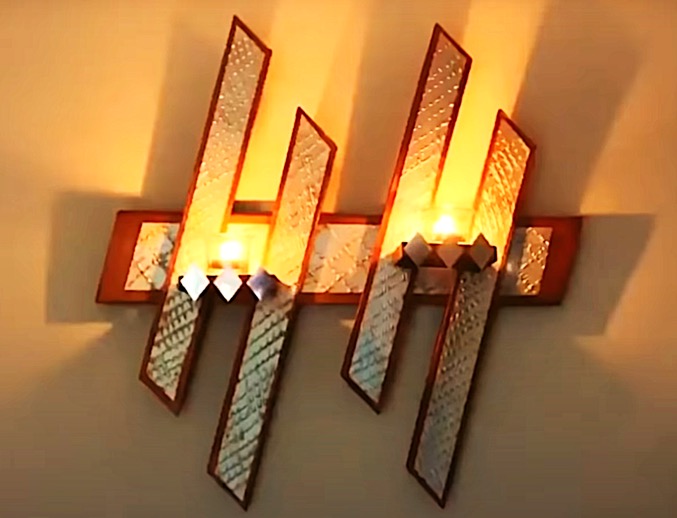The image depicts a rectangular, color photograph taken indoors, featuring an elegantly designed wall light mounted against a deep tan, cream, or orangey-peach colored wall. The wall light consists of a red wooden bar with a gold textured plating at its center, adorned with metallic-like elements that resemble aluminum. Four diagonal or sideways H-shaped metal bars are arranged in pairs next to each other, each embellished with three small diamond shapes. Light emanates from bulbs or possibly lit candles placed above the diamonds, casting a notable luminescence that is reflected on the gold patterns and creating prominent shadows on the wall. The intricate design and interplay of light and shadows give the wall an artistic and sophisticated appearance.